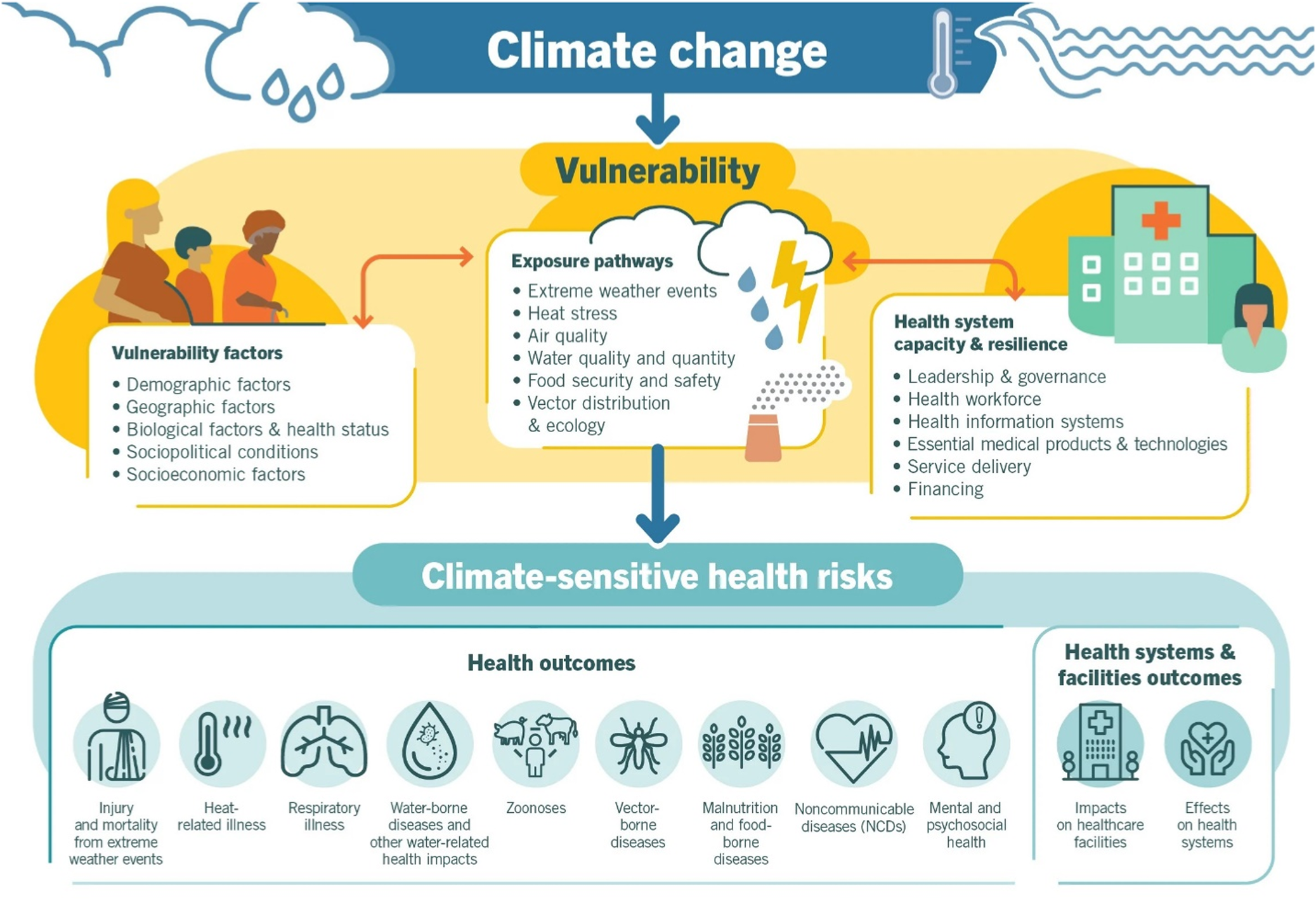The infographic is a horizontally aligned rectangular image on a white background. At the top, there is a blue banner with white text that reads "Climate Change," accompanied by an outline of clouds with raindrops and a thermometer next to ocean waves on the right side. Below, a blue arrow points downwards to a yellow banner with blue text that reads "Vulnerability." Under this, there's a section with the title "Vulnerability Factors," listing demographic factors, geographic factors, biological factors, health status, socio-political conditions, and socio-economic factors. 

A subsequent section titled "Exposure Pathways" includes extreme weather events, heat stress, air quality, water quality and quantity, food security and safety, and vector distribution and ecology. This section features six bullet points. Another arrow points to a section titled "Climate-Sensitive Health Risks" in white text against a green background. 

Further below, a large rectangular area labeled "Health Outcomes" features various circular icons with descriptions. To the right, there's a smaller square area titled "Health Systems and Facilities Outcomes," which contains two circular icons underneath.

On the upper left corner, a cartoon-like illustration depicts three people with varied skin tones and hair colors, and under this, the "Vulnerability Factors" are listed again. On the upper right side, an outline of a hospital with an orange cross is shown, alongside an outline of a woman, under the heading "Health System Capacity and Resilience," followed by six bullet points describing leadership and governance, health workforce, and health information systems.